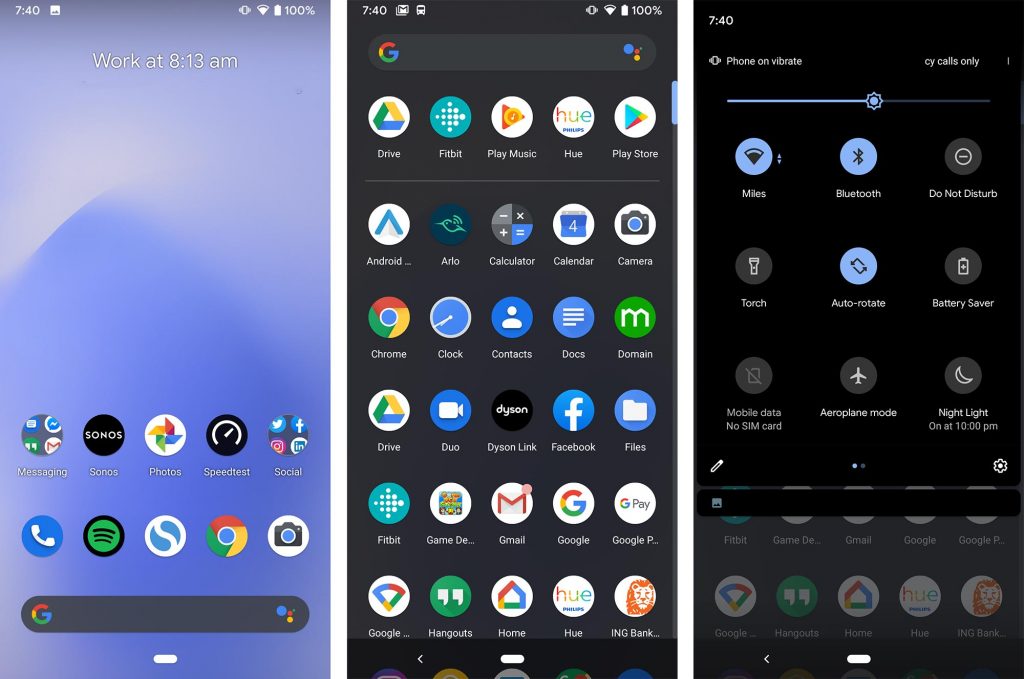Three horizontally aligned screenshots of an Android phone display various settings and apps at 7:40 (either a.m. or p.m.). 

### Image 1:
- **Device Status**: 
  - Silent mode enabled
  - Strong Wi-Fi signal
  - 100% battery
- **Background**: Shades of purple and gray 
- **Notification**: "Work at 8:13 a.m."
  
**Visible Apps**:
- Messages
- Sonos
- Photos
- Speed Test
- Various social apps
- Phone
- Spotify (identified by a white "S" in a blue circle)
- Chrome
- Camera
- Google search bar

### Image 2:
- **Top Usage Apps**:
  - Drive (repeated)
  - Fitbit
  - Play Music
  - Hue
  - Play Store
  - Android apps menu (indicated by "dot dot dot")
  - Arlo
- **Additional Apps**:
  - Calculator, Calendar, Camera, Chrome, Clock, Contacts, Docs, Domain
  - Duo, Dyson Link, Facebook, Files 
  - Fitbit (again), Gaming (identified by "Game, DE, dot dot dot")
  - Gmail (with a notification)
  - Google, Google Pay
  - An indiscernible Google app (resembles a Wi-Fi symbol)
  - Hangouts, Home, Hue
  - ING Bank

### Image 3:
- **Quick Settings Menu**:
  - Vibrate mode enabled
  - Calls only setting for CY 
  - Connected to "Miles Wi-Fi"
  - Bluetooth enabled
  - Do Not Disturb mode off
  - Flashlight off (referred to as "torch")
  - Auto-rotate on
  - Battery saver off
  - Mobile data off (no SIM card detected)
  - Aeroplane mode off
  - Nightlight scheduled for 10 p.m.
  
Additional options include an edit icon (pencil), additional menu dots, and a settings cogwheel, indicating further customization options.

These detailed screenshots reflect various aspects of the user's Android phone, including current status, app usage, and quick settings.